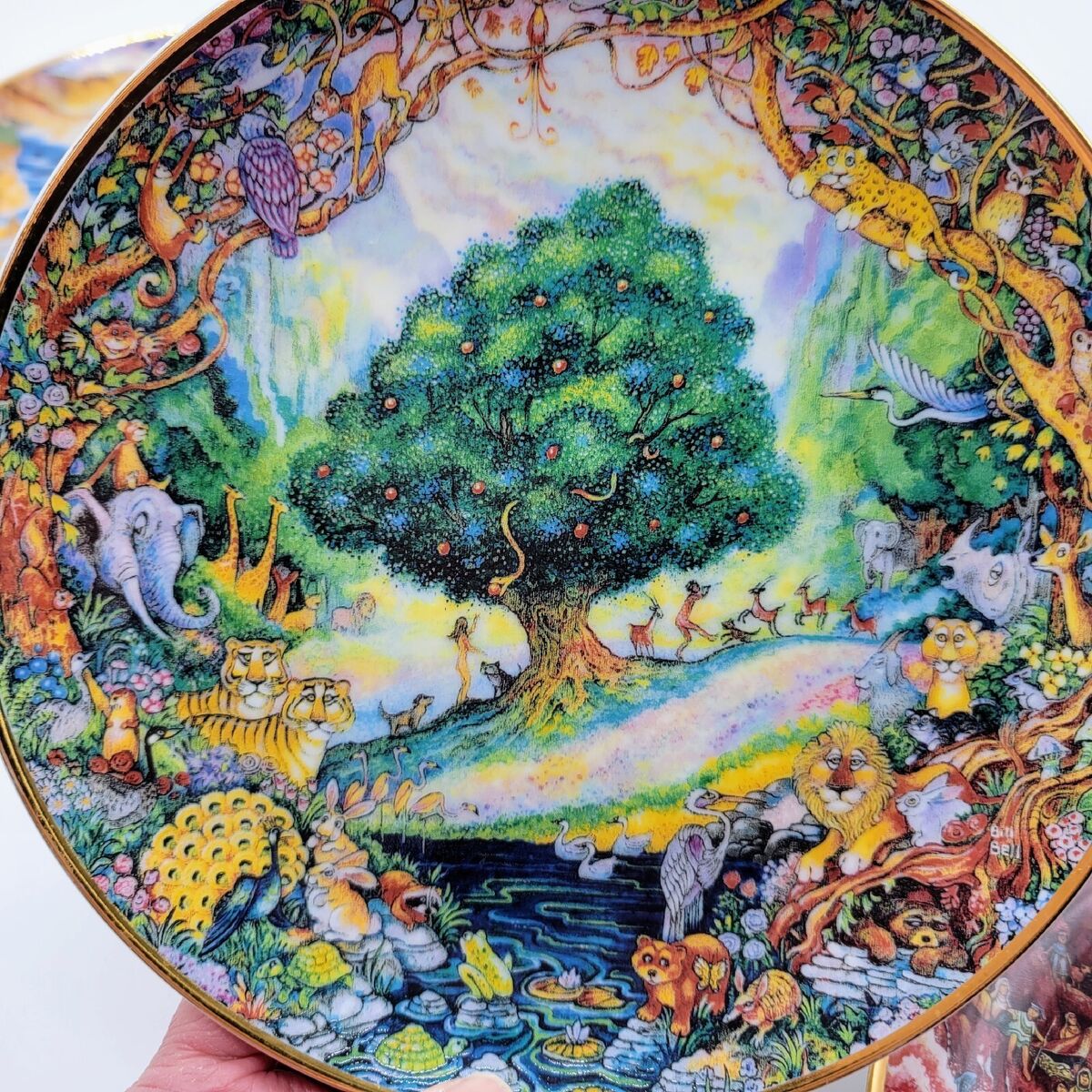This image showcases a beautifully painted, commemorative ceramic plate that illustrates an intricate scene from the Garden of Eden. The central focus is a large, vibrant tree laden with various fruits, where a snake can be seen offering an apple to a naked Eve, who reaches up to take it. To the right, a naked Adam appears to be playing a flute, serenading a group of animals that include deers and gazelles. Surrounding the central scene, the plate features a diverse array of animals rendered in a charming, almost cartoon-like style. Among these are turkeys, bears, lions, elephants, monkeys, an owl, and a vulture, all depicted against a backdrop of vines and trees. The overall color palette is rich and varied, featuring shades of yellow, green, red, brown, and orange, indicative of the artist's attention to detail and dedication. The plate is being held up by a person, with their hand and thumb visible in the image. In the background, additional painted plates can be observed, adding depth and context to the scene. This meticulous work of art highlights both the mythical narrative and the artist's extraordinary craftsmanship.